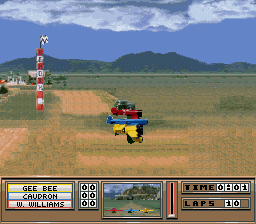This image is a screenshot from an older-style video game, which features a blend of pixelated and slightly 3D visuals. The main focus of the scene is a red tractor-like object situated in a vast open field, seemingly engaged in a race. Below it, there's a smaller yellow tractor or piece of farm equipment. To the right of these tractors, a slender blue vehicle, possibly an airplane, is noticeable, suggesting a multi-vehicle race scenario. 

The lower portion of the screen displays various control panels and screens, potentially showing the game’s interface or an airplane simulator's dashboard. The right side of the screen includes time slots and lap counts, while the left side features additional statistics, likely representing the different players competing in the game. 

A red and white stack tower with the word "Welcome" and a waving checkered racing flag enhance the race atmosphere. Despite the small image size making details challenging to discern, the combination of the red, yellow, and blue vehicles, along with the surrounding elements, vividly illustrates a competitive race setting in this pixelated game environment.